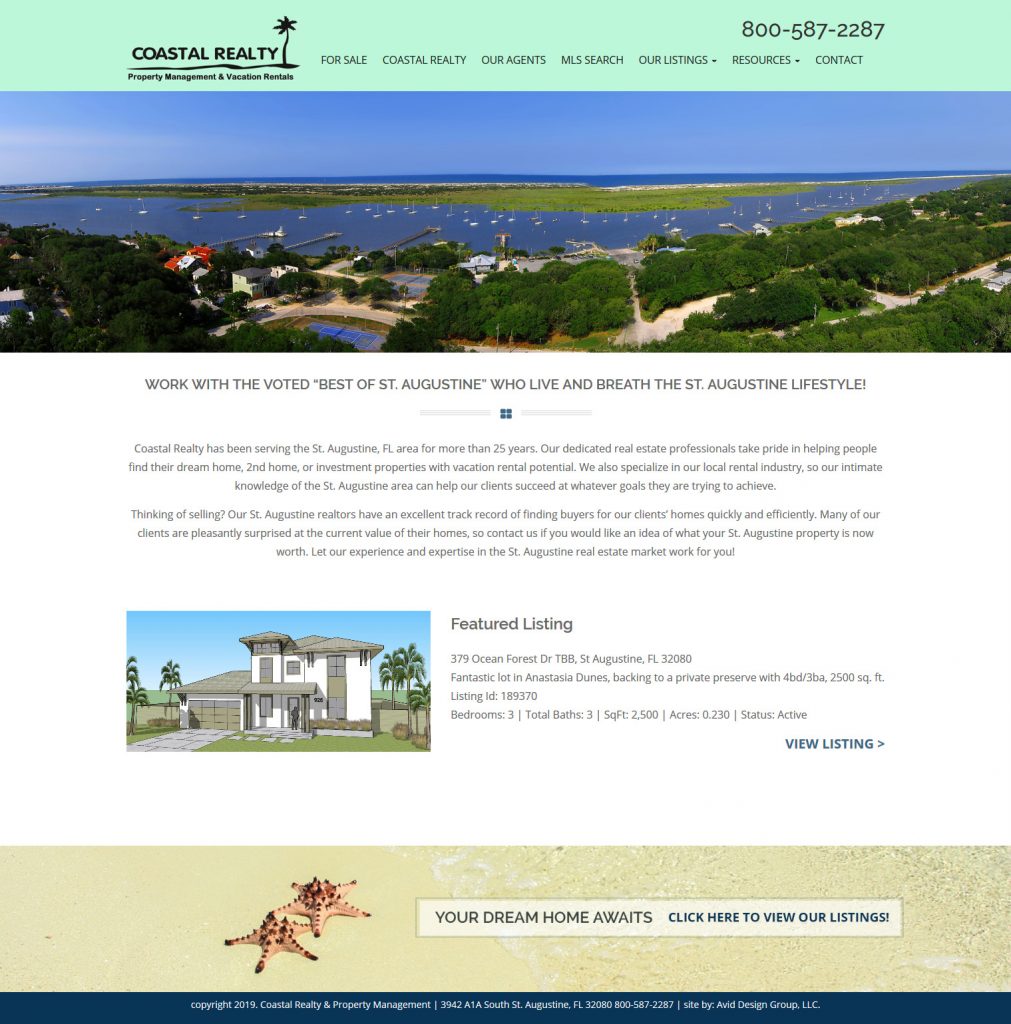This web page belongs to Coastal Realty and features a stunning banner photo of a picturesque shoreline and beach in St. Augustine, Florida. Highlighted prominently on the page is a featured listing for 379 Ocean Forest Drive, St. Augustine, Florida, though the price is not displayed. The site includes general information about the realtor group, although the text is too small to read clearly. Navigation tabs at the top of the page guide users to sections such as 'For Sale,' 'Coastal Realty,' 'Our Agents,' 'MLS Search,' 'Our Listings,' 'Resources,' and 'Contact.' For inquiries, the contact phone number is 1-800-587-2287.